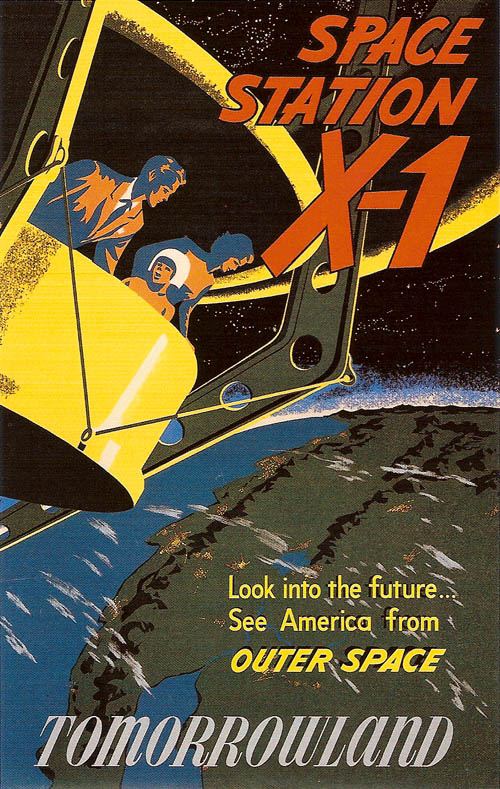This hand-drawn, vintage advertisement, styled like a comic book cover, is for "Space Station X1." At the top right, bold red letters proclaim "Space Station X1" with the "X1" prominently large. In the upper left, a family—a man, a woman, and a child—are depicted gazing out from a yellow or green viewing platform that resembles a hot air balloon basket or a Ferris wheel bucket, suspended in outer space. This platform offers a stunning view of Earth below, specifically highlighting the Baja Peninsula and North America. The background sky is black, emphasizing the vastness of space. Below the primary title, in vibrant yellow font, the caption reads "Look into the future. See America from outer space," with "outer space" capitalized for emphasis. At the very bottom, in light gray, the word "Tomorrowland" indicates a futuristic theme park attraction or vision. This imaginative ad invites viewers to dream of a future where families can enjoy thrilling views of Earth from a space station.